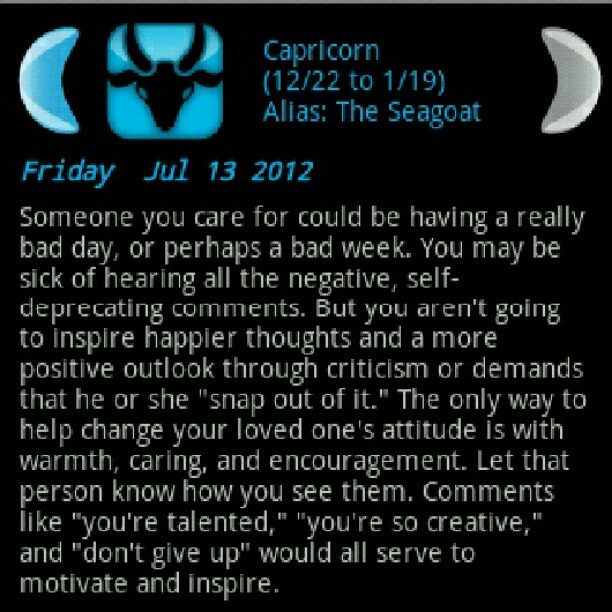The image depicts an online horoscope for the Zodiac sign Capricorn, dated Friday, July 13, 2012. In the top left corner, there are navigation arrows; a rounded blue arrow pointing left and a rounded gray arrow pointing right, suggesting the ability to scroll through different Zodiac signs. Next to the left arrow is a bright blue square icon with a black silhouette of a goat, symbolizing Capricorn. Below this, the text "Capricorn 12/22 to 1/19 alias the Seagoat" is displayed. The horoscope message reads: "Someone you care for could be having a really bad day or perhaps a bad week. You may be sick of hearing all the negative, self-deprecating comments, but you aren't going to inspire happier thoughts and a more positive outlook through criticism or demands that he or she snap out of it. The only way to help change your loved one's attitude is with warmth, caring, and encouragement. Let that person know how you see them. Comments like, 'You're talented,' 'You're so creative,' and 'Don't give up,' would all serve to motivate and inspire."